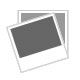The image displays a brightly lit belt with a looped structure, appearing to be made from a material resembling weathered leather or suede. The outer side of the belt features a light beige, almost grayish hue, while the inner side is more distinctly taupe or light brown. The belt's detailed stitching runs across the entire loop, adding texture and definition. At the front, the belt fastens with a unique buckle consisting of two rectangular silver pieces, possibly magnetic, each adorned with a hammered design featuring rows of small, indented circles. The belt has a plush and padded appearance, suggesting a soft, cushioned texture, emphasizing its thick and plush construction. The white background of the photograph highlights the three-dimensional aspects and subtle details of the belt.